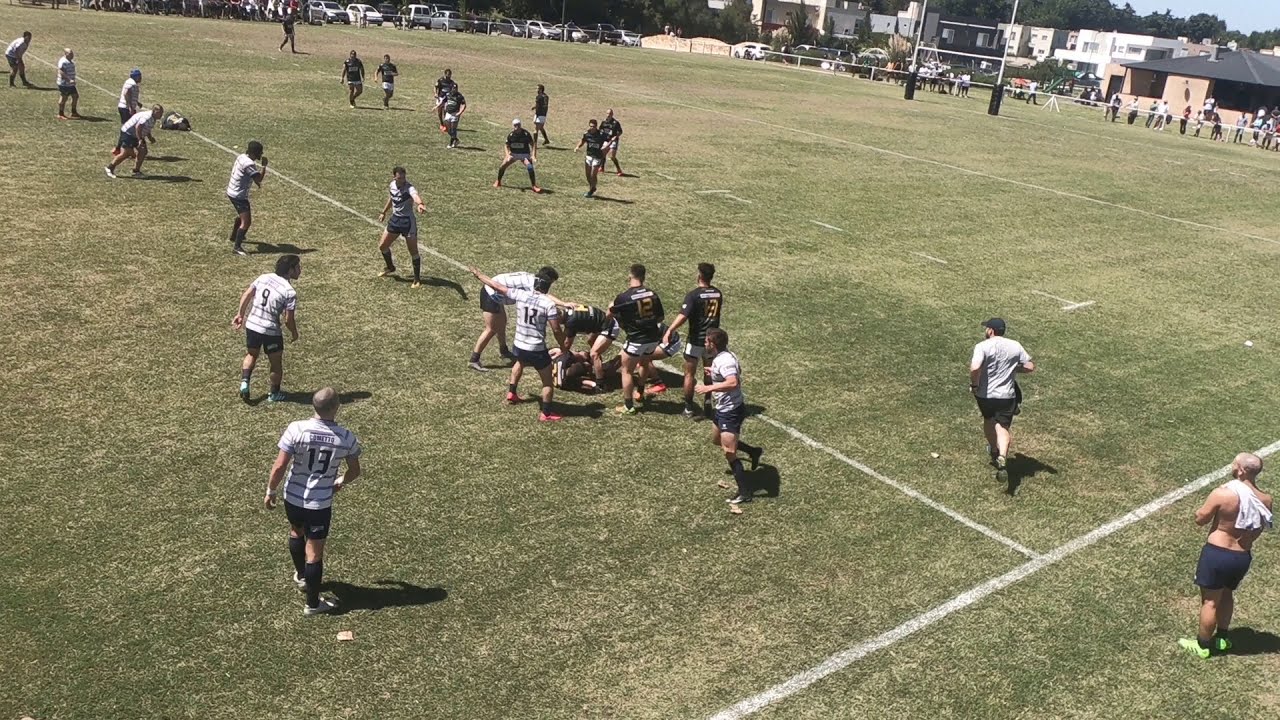The image captures a diagonally angled, wide rectangular view of a neatly trimmed grass field where a group of people appears to be playing rugby or possibly a form of football, as evidenced by the goalposts visible in the distance. The players are divided into two teams: one team in white striped shirts positioned on the left side of the image, lining up in a row, and another team in black shirts located closer to the top of the image. The perspective reveals much of the field, with white sideline paint partially visible crossing the bottom right corner. The horizon line, which slopes slightly downward to the right, reveals several buildings of various colors and a parking lot filled with cars. Additionally, a concession stand is located at one end of the field, possibly surrounded by onlookers or fans. There appears to be some potential action or commotion towards the middle of the field, as one player is on the ground, seemingly surrounded by teammates.